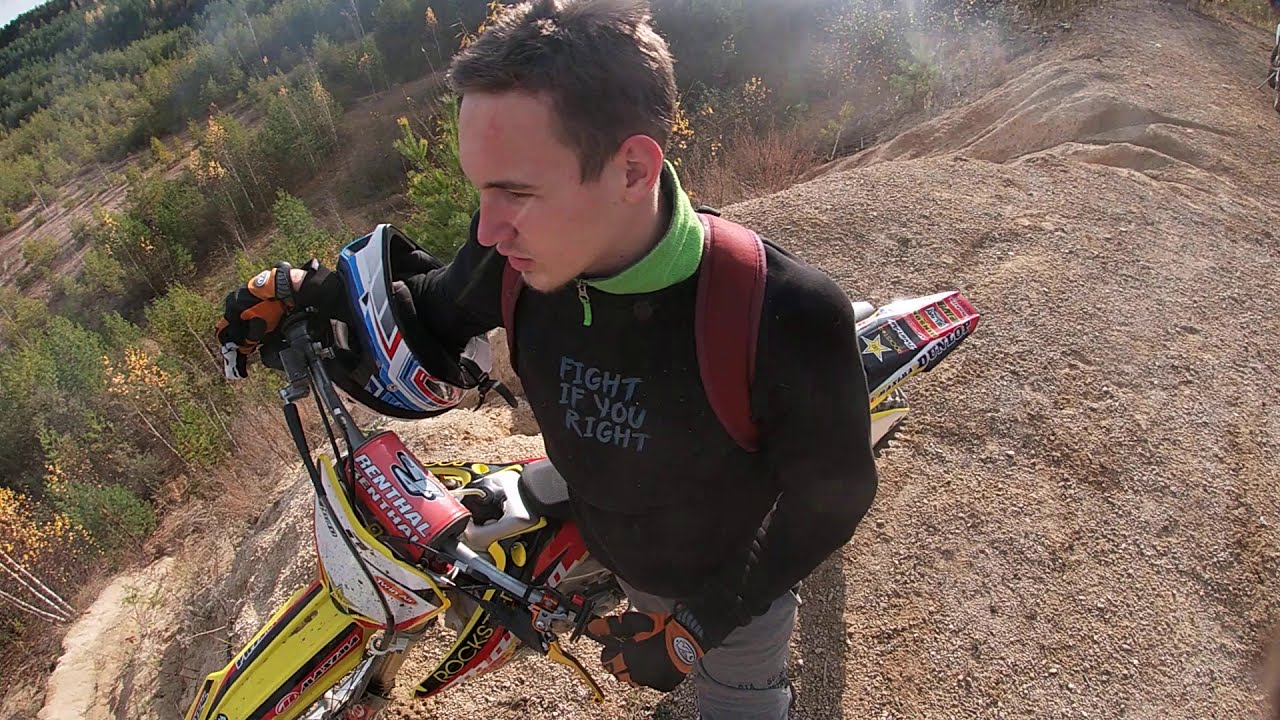This image captures a detailed outdoor scene taken during daylight, featuring a young Caucasian man positioned on the edge of a rocky cliff or grey stone promontory. The photo is shot from an elevated angle, providing a top-down view of the subject. He has short brown hair and a hint of stubble on his chin. His attire includes a black long-sleeved shirt with a green collar and the phrase "FIGHT IF YOU WRITE" emblazoned in gray, casual, handwritten-style capital letters on the front. Over this, he wears a red-strapped backpack.

The man is holding the handlebars of a small yellow dirt bike with a varied color scheme of yellow, black, and red. The brand name "Renthal" is prominently displayed twice in white letters on the red section at the center of the handlebars. He has his right arm threaded through a full-face helmet — which is predominantly white with red, blue, and black details — letting it hang from his arm. He's also wearing orange and black gloves. 

The cliff edge he stands on is smooth, and it drops sharply into a valley filled with green trees and scattered dirt patches below. The landscape transitions from thin pine trees in the foreground to a denser forest of darker trees in the background. The photographer captures him looking straight ahead, standing at the very edge of this natural precipice, giving a sense of both tranquility and adventure.